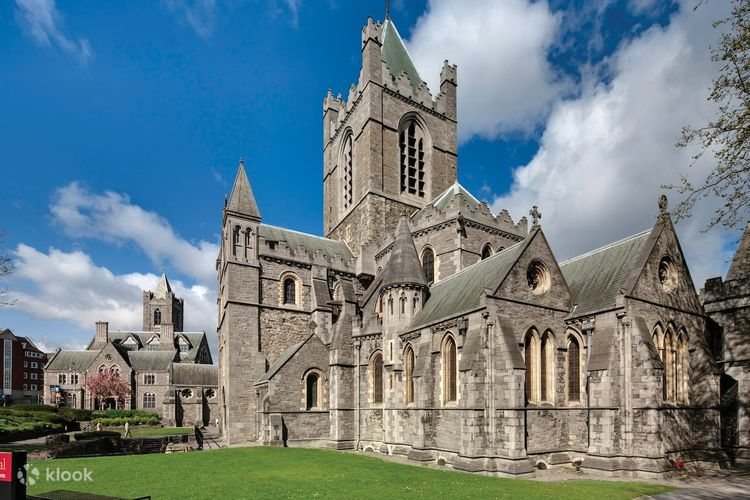The image is a landscape color photograph capturing a historic gothic church made of stone, believed to be several hundred years old. Taken from the rear of the church, the photograph showcases the most prominent side, which features towering turrets, steeply pointed roofs, and arched stained glass windows, including rose windows at the top of the gables. The background is a bright blue sky with a few clouds, emphasizing the sunny and clear day. 

In the foreground, a finely manicured green lawn stretches out, devoid of any shrubs or weeds, providing a clean, well-kept appearance. On the left-hand side of the image, a blossoming tree with pretty pink petals adds a touch of color and vibrancy. Additionally, a waterway is visible in this corner, enhancing the serene atmosphere of the scene. 

Interestingly, the church is part of a larger religious compound, as indicated by the presence of another equally aged stone church in the background, possibly connected by stone buildings. Two people can be seen walking in the courtyard, adding a sense of scale and life to the historical setting. The image also features a brand name, "Kluk," along with their logo in the bottom left corner. Overall, the photograph captures the beautiful architecture, rich history, and serene surroundings of this impressive gothic church.